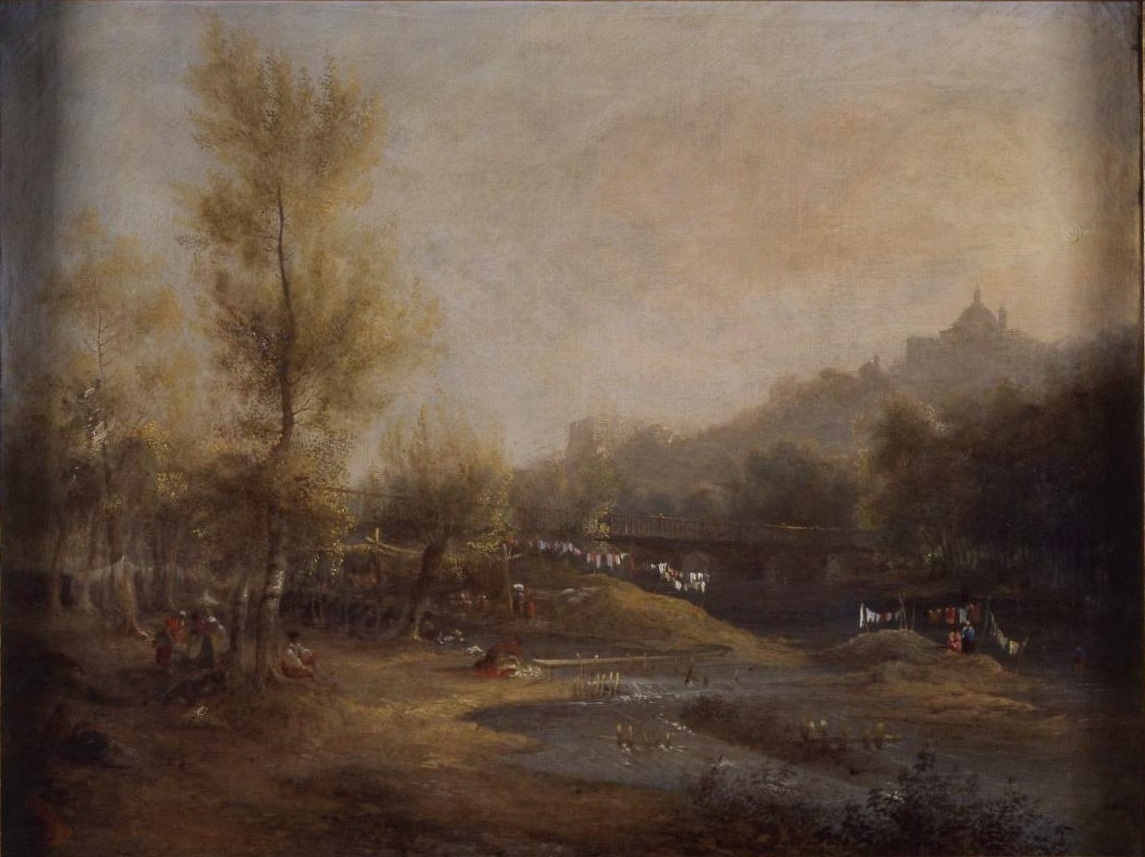The painting depicts a serene, late 19th-century countryside scene on the outskirts of town. The upper half of the image is dominated by a hazy light blue sky with faint clouds, complemented by hints of peach and beige. Below, a river meanders through a flat landscape, flowing under a bridge towards a striking hill in the background. This hill is crowned with a domed building and what appears to be a castle-like structure. The foreground is lively with dense foliage—trees painted in grayish-green tones—and a bank lined with grass and trampled dirt.

In the immediate foreground, the daily life of the inhabitants unfolds. Several clotheslines, tethered between thin poles, display freshly washed clothing, blowing gently in the breeze. Women are seen lounging on blankets, enjoying the sunny day, while other villagers mill about near the trees. A man sits in the shade under a tall tree on the left, which reaches from the bottom left corner to the top of the image. 

The left side is densely wooded, while the right side shows more sporadic trees interspersed along the riverbank, creating a picturesque balance in the described rustic setting. The scene is characterized by its muted colors and low contrast, evoking the simplicity and tranquility of early rural life.